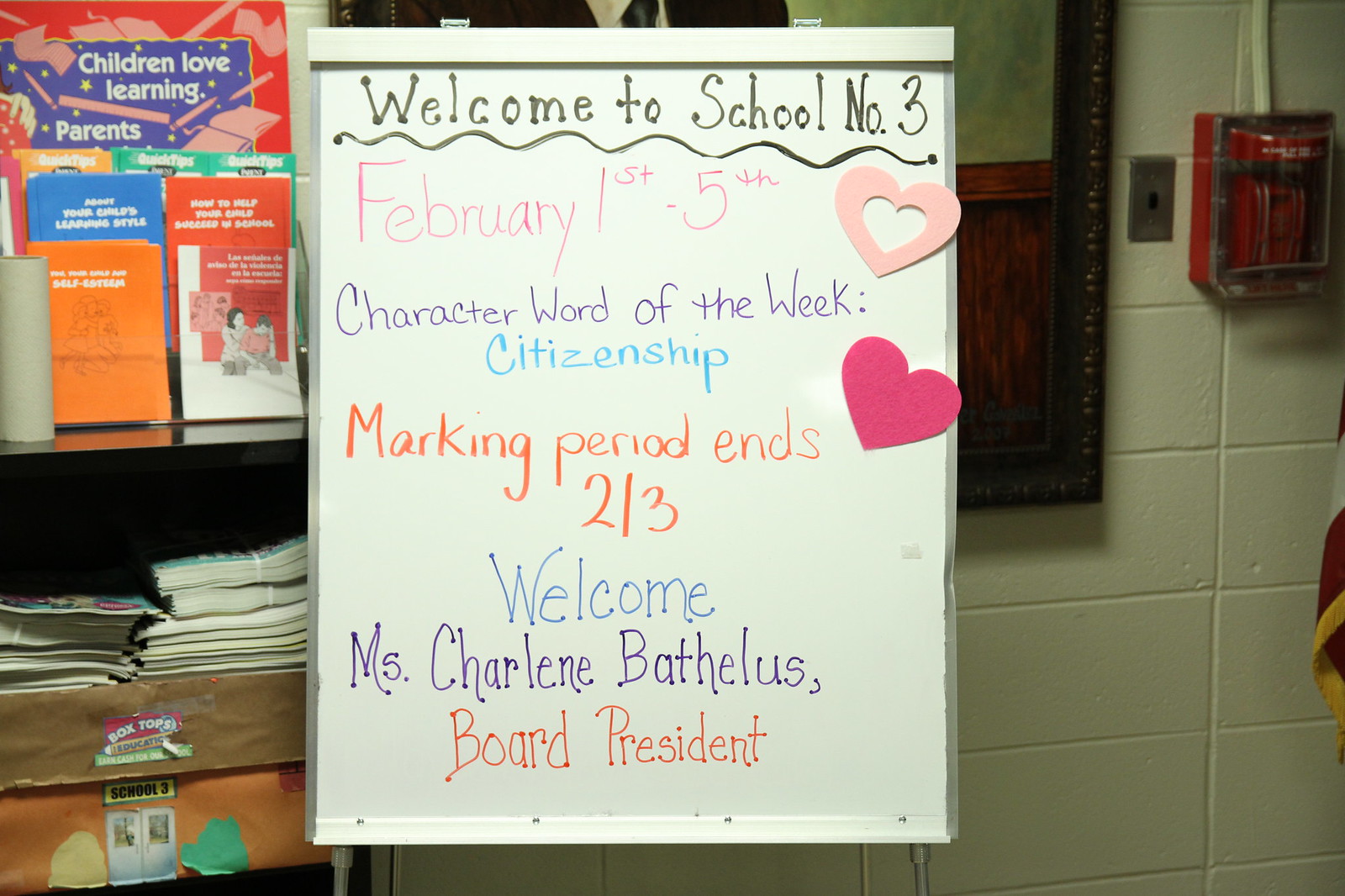The photograph captures a vibrant classroom setting with a white stone wall in the background, featuring a whiteboard sign on a silver easel at the center. The sign, written in various colors, welcomes students to School Number Three and features several important notices. The message, handwritten in green and black markers, reads: "Welcome to School Number Three," with a squiggly line underneath. In pink, it displays the dates "February 1st - 5th." To the right, two construction paper hearts are taped, adding a touch of creativity and warmth. The sign also highlights the "Character Word of the Week: Citizenship" in blue, the "Marking Period Ends 2-3" in orange, and a cheerful "Welcome" followed by "Miss Charlene Bathelis, Board President" in a girly font. On the right side of the image, a fire alarm with a plastic cover is mounted on the wall. To the left, a small shelf holds brochures and a "Box Tops for Education" display, with the top shelf labeled "Children Love Learning."